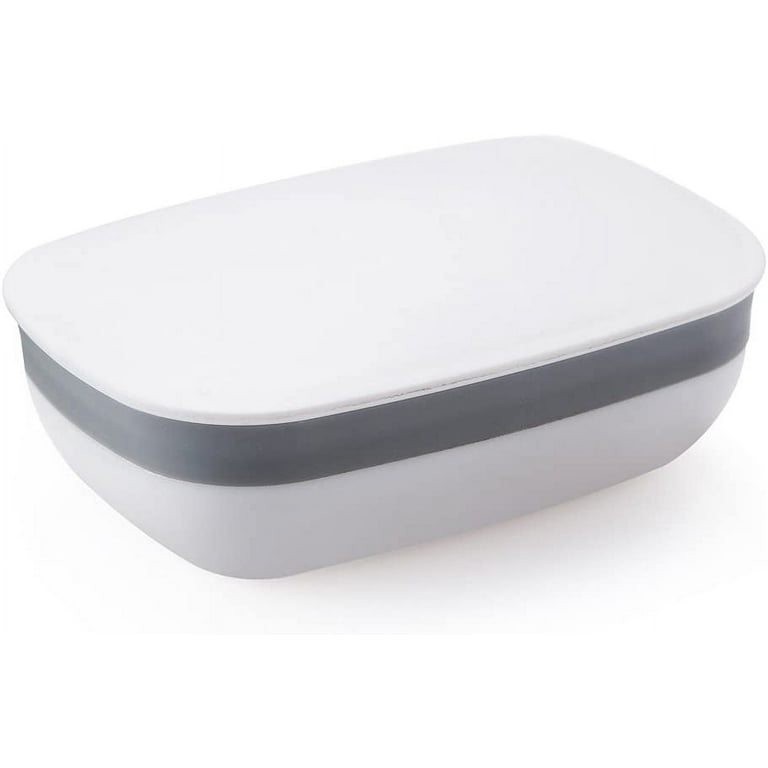The image displays a simple, plain plastic container set against a solid white background. The container is primarily off-white in color and features a prominent gray band around its top edge, just beneath a tightly fitted white lid. Its rounded corners and elongated shape suggest versatility in storage, fitting easily into a refrigerator or on a shelf. The container, which is devoid of any branding, logos, or designs, appears to be a generic Tupperware-like item that could be used for preserving food, leftovers, or marinating ingredients. The absence of any reference objects or scale makes it difficult to determine its exact size, leaving it ambiguous whether it is a small butter dish or a larger item suitable for casseroles.